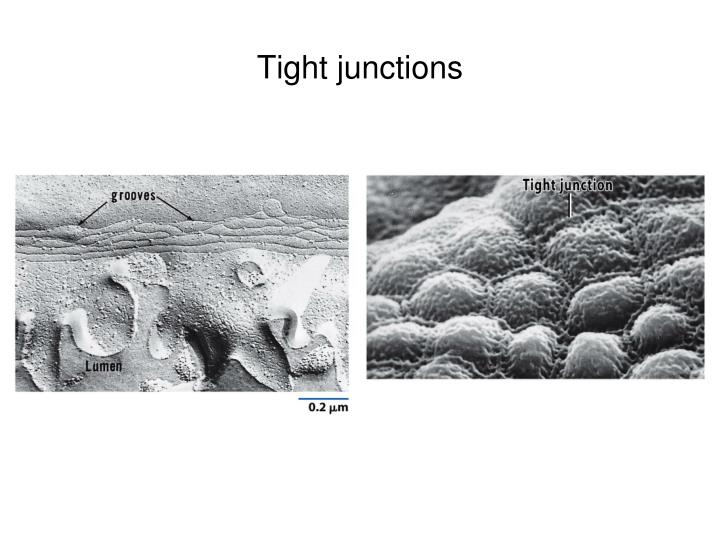The image is titled "Tight Junctions" in bold, black text at the top and showcases two different microscopic views side-by-side on a white background. The left-hand image, resembling a textured black and white surface akin to a lunar landscape, includes labeled regions with arrows: "grooves" and "lumen." This image appears to offer a multi-layered view at a microscopic level, where the grooves indicate the locations of tight junctions within this context. Additionally, there is a size scale in the lower right corner of this image, providing a sense of scale. The right-hand image, also black and white and featuring a lumpy texture, identifies a specific tight junction with an arrow and label. Together, these images provide both a detailed cross-sectional look at tight junctions on the left and a broader, less detailed view on the right, enhancing the understanding of their structure and positioning.